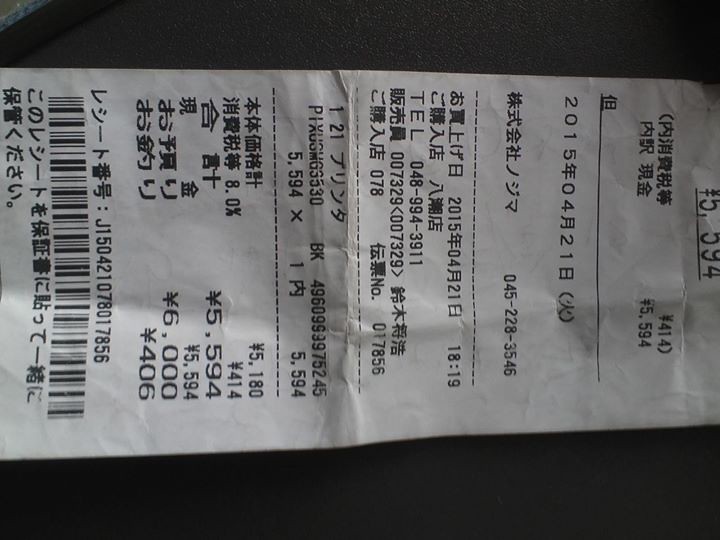This image is a colored photograph of a close-up receipt in Japanese. The photograph is rotated 90 degrees to the right, positioning the text vertically from the left or the top to the bottom rather than the conventional left to right. The receipt features numerous Japanese characters, indicating various line items with their respective amounts: 5,154 yen, 400 yen, and 5,594 yen, with the total summing up to 6,000 yen. A date is also visible, formatted in numerals as 2015-04-21. Additionally, there's a telephone number printed in Roman numerals, "TEL 048-994-311", centered on the receipt. The receipt appears to be white against a black background, and there is a barcode visible on one side. This detailed receipt suggests a substantial amount was spent, possibly in a restaurant or similar establishment.